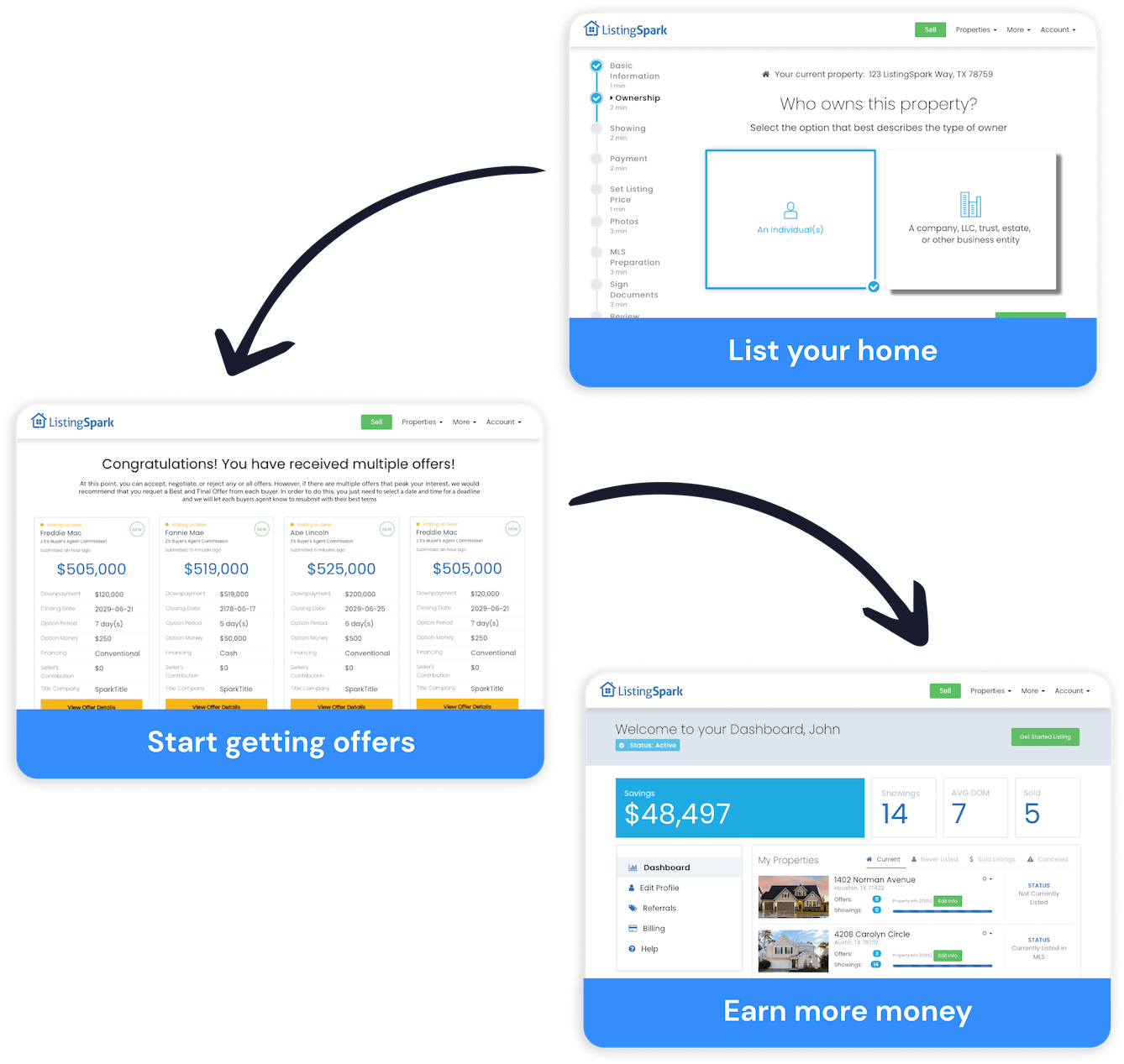This image consists of three interconnected rectangles forming a flowchart, each linked by arrows depicting a guided process. 

At the very top, the first rectangle is titled "Listing Spark" and includes checkmarks next to the steps "Basic" and "Ownership," indicating completed stages. Within this rectangle, details about the current property are listed, including the address and zip code. The user is prompted to select the type of owner for the property, with "Individual" being highlighted, while other options such as "Company," "Trust," and "Estate" are also available but not selected.

An arrow from this first rectangle points downward to the second, positioned towards the left. This rectangle is titled "List Your Home." It features a congratulatory message indicating that multiple offers have been received for the property, with offers ranging from $505,000 to $555,000. Below this information, there's a call-to-action button labeled "Start Getting Offers."

Another arrow leads from this second rectangle to the final one at the bottom center of the image. Here, the rectangle is labeled "Earn More Money," featuring a welcoming message that reads, "Welcome to your dashboard, John."

The image effectively guides viewers through the steps involved in listing a property, receiving offers, and accessing the dashboard for further actions.